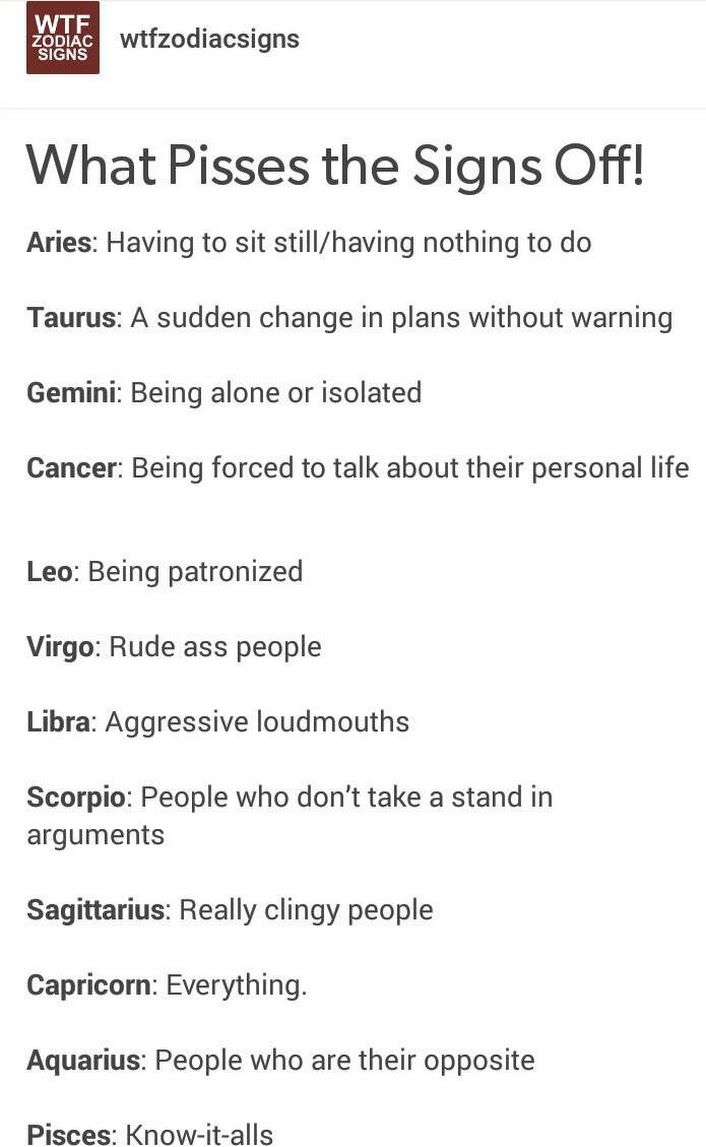The image is a detailed infographic on a plain white background, centered around Zodiac signs. In the upper left-hand corner, there's a maroon square logo with "WTF" on the first line, "Zodiac" on the second, and "Signs" on the third, all in white text. Next to the logo, the company name, "WTFZodiacSigns," is written in black text. The infographic is titled "What Pisses the Signs Off!" in large black font. Below the title, each Zodiac sign is listed in bold with their respective pet peeve detailed in regular font. The list reads as follows:

- Aries: Having to sit still / having nothing to do
- Taurus: A sudden change in plans without warning
- Gemini: Being alone or isolated
- Cancer: Being forced to talk about their personal life
- Leo: Being patronized
- Virgo: Rude-ass people
- Libra: Aggressive loudmouths
- Scorpio: People who don't take a stand in arguments
- Sagittarius: Really clingy people
- Capricorn: Everything
- Aquarius: People who are their opposite
- Pisces: Know-it-alls